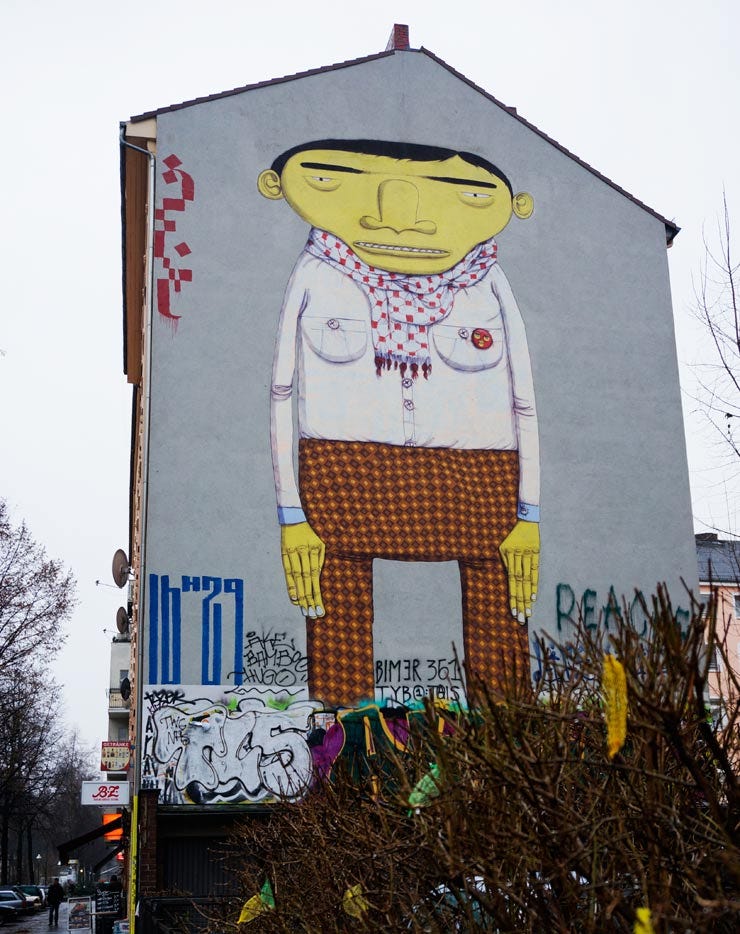The image captures the side of a gray building, possibly a house or business, adorned with a detailed mural. The centerpiece of the mural is a stylized, wide-faced man with yellow skin, short black hair, small ears, a wide nose, and a narrow mouth with eyes set far apart. He wears a form-fitting white shirt with buttons positioned where his nipples would be, one of which is red and on the left pocket. Around his neck is a white scarf with red squares, and he dons 70s-style checkered pants, orange-brown with red and yellow blocks. Amidst the artwork, there are various graffiti elements, including abstract shapes, the characters 16H29, and TG5 or TGS, with some graffiti partially concealed by a dead bush in the foreground. To the left, there are indications of a street with people, cars, signs, and trees, set against an overcast sky.